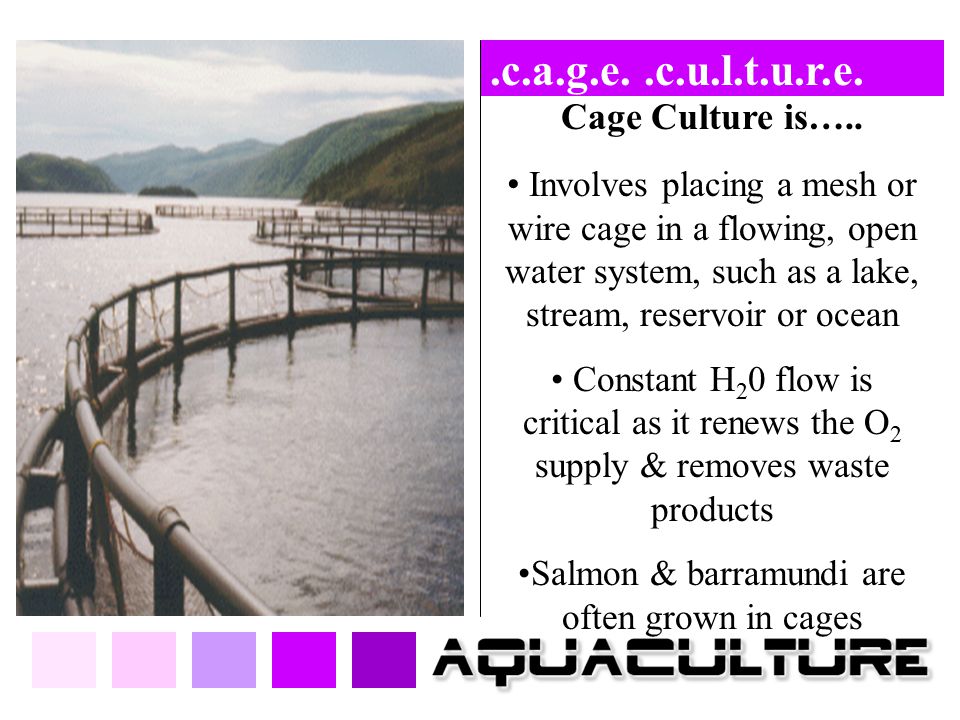The image is a colorful educational infographic focused on "CAGE CULTURE." On the left side of the infographic, there is a somewhat dull, gray-toned photograph featuring a body of water with six circular cage structures arranged in it, likely used for aquaculture fish farming. In the background, rolling hills with shades of green and brown add depth to the scene. To the right of the photograph, the infographic includes detailed text, starting with a purple rectangle containing white letters that spell "CAGE CULTURE." Below that, in black letters, "CAGE CULTURE IS" serves as a heading for three informative bullet points: 

1. Involves placing a mesh or wire cage in a flowing open water system such as a lake, stream, reservoir, or ocean.
2. Constant H2O flow is critical as it renews the O2 supply and removes waste products.
3. Salmon and barramundi are often grown in cages.

Beneath the text, there is a sequence of five squares, transitioning from light pink to dark purple, adding a visual gradient. At the very bottom, bold black letters spell "AQUACULTURE," emphasizing the focus of the infographic. Overall, the layout and color scheme give the infographic an educational feel, clearly designed to convey information effectively.